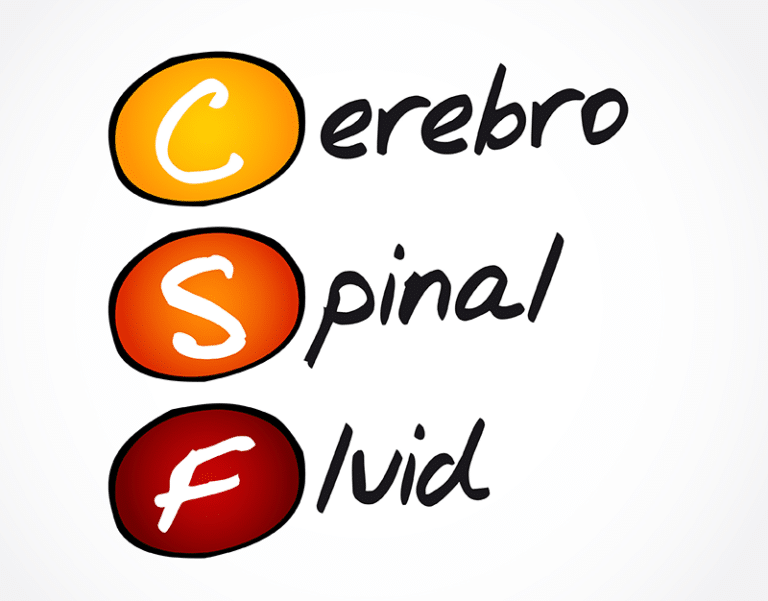This image displays a rectangular, light gray digital graphic featuring the acronym for "Cerebrospinal Fluid." The text is arranged in three rows, each beginning with a large white letter inside a colored circle, followed by the remaining letters of the word in black lowercase. The first row starts with a white "C" enclosed in a yellow circle, followed by "erebro." The second row includes a white "S" within an orange circle, followed by "pinal." The third row shows a white "F" inside a red circle, followed by "luid." This creative and cartoonish design contrasts the serious nature of the term "cerebrospinal fluid," giving it a playful visual twist.